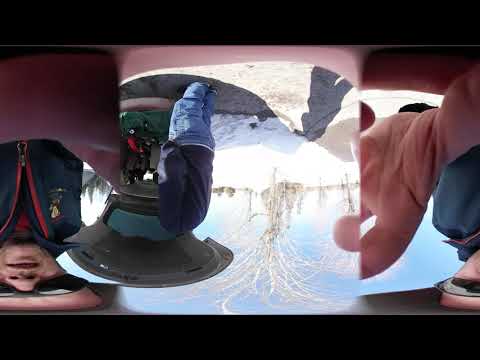The image appears to be a heavily Photoshopped or edited composite that is vertically rectangular with thick horizontal black stripes across the top and bottom. The image displays three distinct sections: 

On the left, there is an upside-down view of a person, visible from the waist up, wearing a dark blue shirt or hoodie, black sunglasses, and possibly a black coat with a red zipper. Their proportions appear distorted, indicating the use of a specialized lens or editing technique.

In the center, another upside-down image shows an outdoor scene with bare trees and snow-covered ground, hinting at a winter setting. There is an individual standing with their back to the camera, clad in a navy blue jacket and jeans. Above their head is a machine-like object or some equipment, adding to the surreal atmosphere.

On the right side, the picture shows a person's leg and foot on the ground in a sideways position. This person is also wearing a black upper garment and black sunglasses. Part of their arm is visible, and they seem to be interacting with the camera in some way.

Altogether, these elements combine to create an image that defies logical interpretation, characterized by its inverted and distorted representations of people and outdoor scenery.